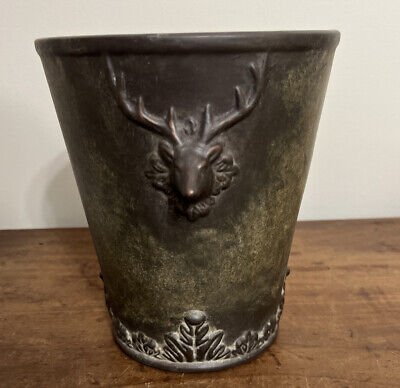A vintage, cast iron bucket is centrally positioned in the image, facing directly towards the camera. Constructed from a dark, robust metal reminiscent of cast iron, the bucket features a flared design—wider at the open top and gradually tapering towards the narrower base. The bucket rests on a high-quality wooden floor, which adds a rustic charm to the scene. The base of the bucket is adorned with an intricate leaf pattern that seamlessly blends with its overall color, maintaining a cohesive, monochromatic look. Dominating the center of the bucket's front is a meticulously crafted moose head, projecting outward and adding a touch of elaborate detail and character to this otherwise utilitarian object.